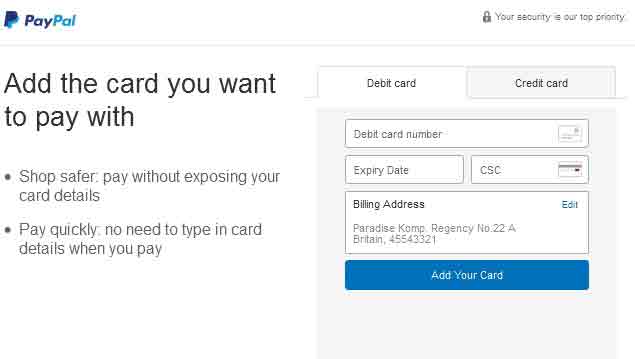This image is a screenshot from the PayPal website, and the background is predominantly white. In the upper left corner, the PayPal logo is displayed: "Pay" is written in a navy blue font, and "Pal" is written in a sky blue font. To the left of the text, the letter "P" is formed with a navy blue color and a sky blue shadow effect beneath it.

At the top right of the image, there is a gray padlock symbol accompanied by the text "Your security is our top priority." On the left side, a prominent message in large gray font reads, "Add the card you want to pay with." Below this message, there are two bullet points:
1. Shop safer, pay without exposing your card details.
2. Pay quickly, no need to type in card details when you pay.

On the right side of the image, there is a rectangular section with two tabs at the top. The "Debit Card" tab is highlighted with a white background, while the "Credit Card" tab has a very light gray background. Below these tabs is a form for inputting debit card details. The form includes:
- A rectangle for the debit card number.
- A section beneath that for the expiration date, followed by an area for the CSC (the three-digit code on the back of the card).

Further down, there's a large rectangle labeled "Billing Address." To the right of this label, "Edit" is displayed in blue font. An example billing address is pre-filled in the form: "Paradise Comp, KOMP Regency, 22-A Britain, 45543321."

At the bottom of the form is a blue rectangle button with white text that reads "Add Your Card," indicating the action to complete the input process.